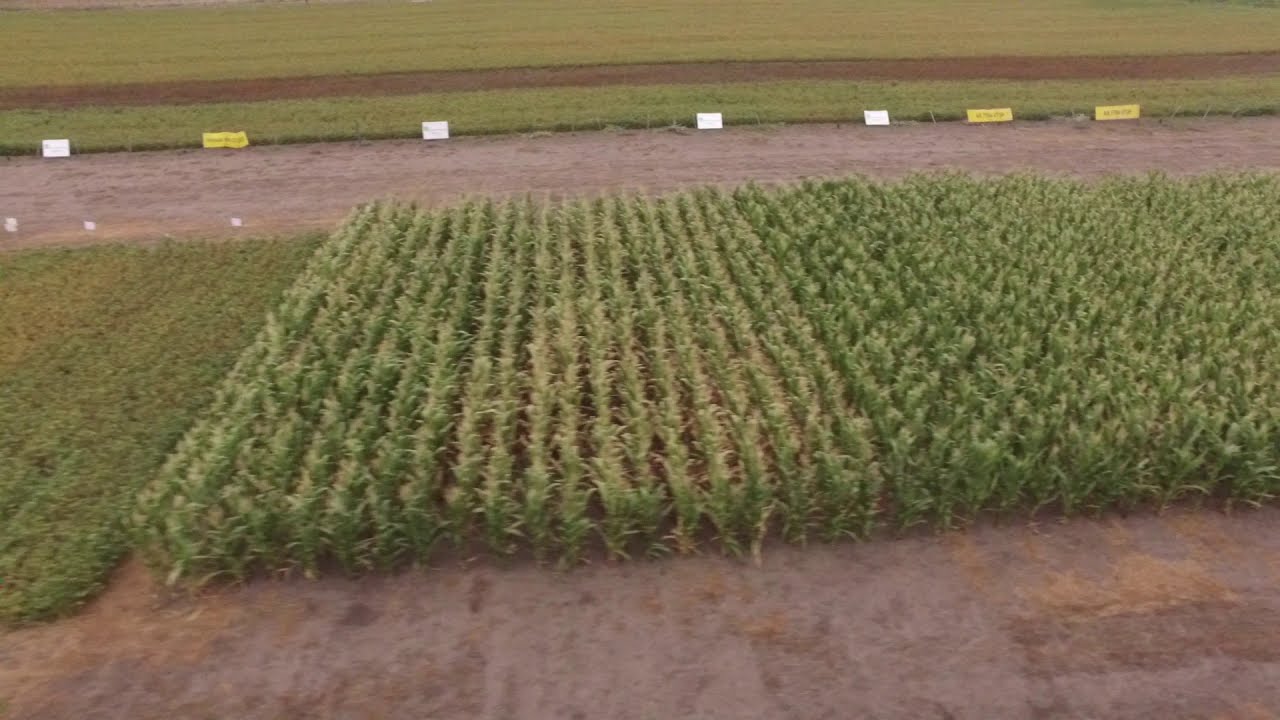This aerial view of a farmland scene depicts a well-organized agricultural setting. The central focus is on numerous rows of green crops, likely corn, stretching horizontally across the image. To the left of these rows, there are patches of short, low-lying plants. The background showcases an expanse of lush green grass. Framing the crops, there are two dirt paths resembling roadways—one in front and one behind the planted rows—both smoothed and flattened, providing clear separation from the crops.

Lining the edge between the front dirt path and the crops, there are several rectangular signs laid out in an identifiable pattern: starting with a white sign, followed by a yellow one, then three consecutive white signs, and finally two yellow signs. While the writing on these signs is not legible, they punctuate the landscape prominently. Overall, the image vividly captures the orderly beauty and structured division of agricultural fields.